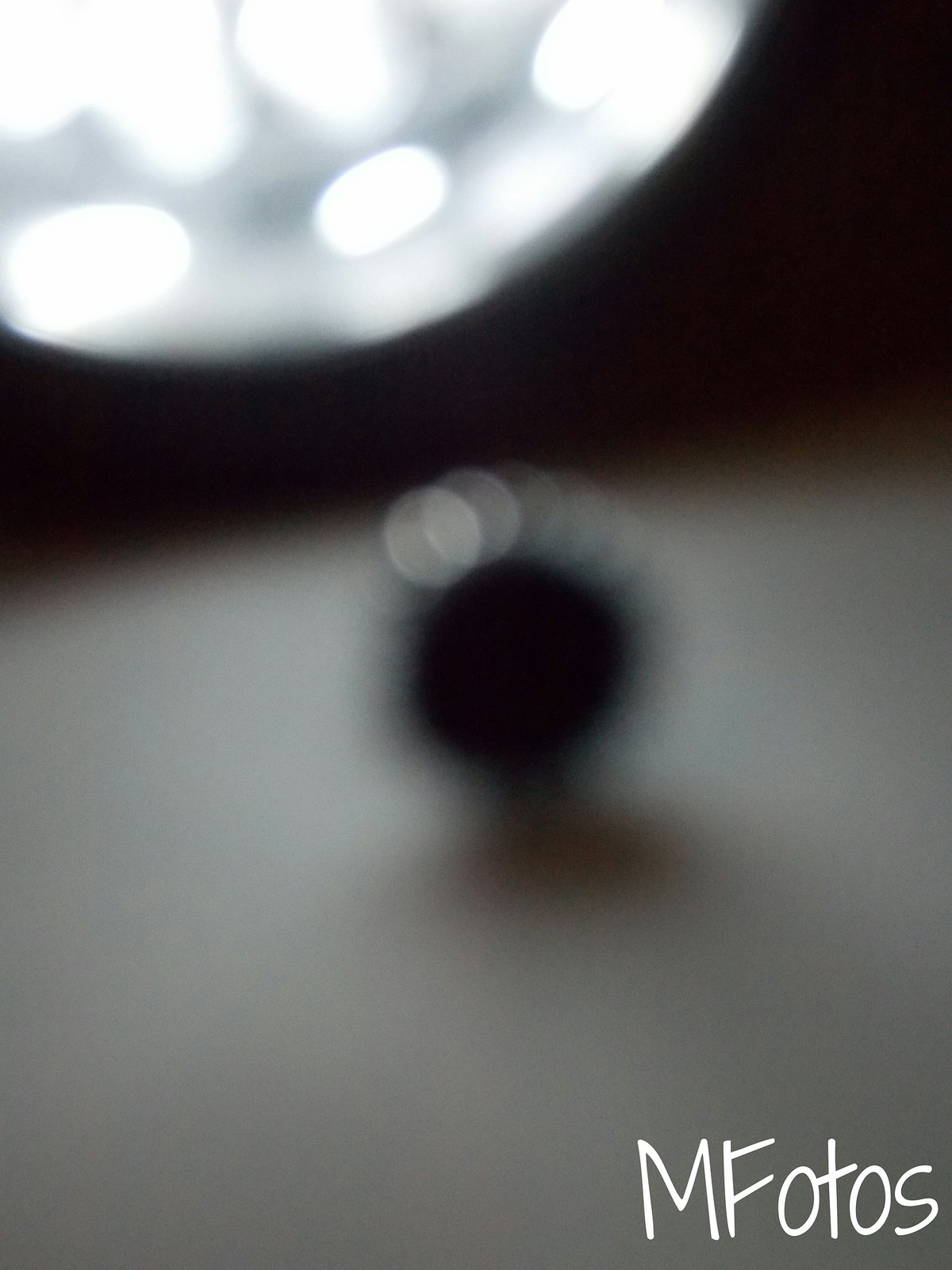This image depicts a blurry, round dark object positioned centrally, surrounded by small light circles, likely reflections from a physical light bulb. The object rests on an indistinct light-colored surface, possibly beige. Above this, there is a horizontal section stretching across the image from left to right that is dark brown, almost black. Further up, a partially visible white half-circle with gray patches and approximately seven brighter white spots extends off the edge of the picture. In the bottom right corner, the letters "M Photos" appear, with "M" and "P" as capitals and the rest in lowercase, suggesting a watermark or label.